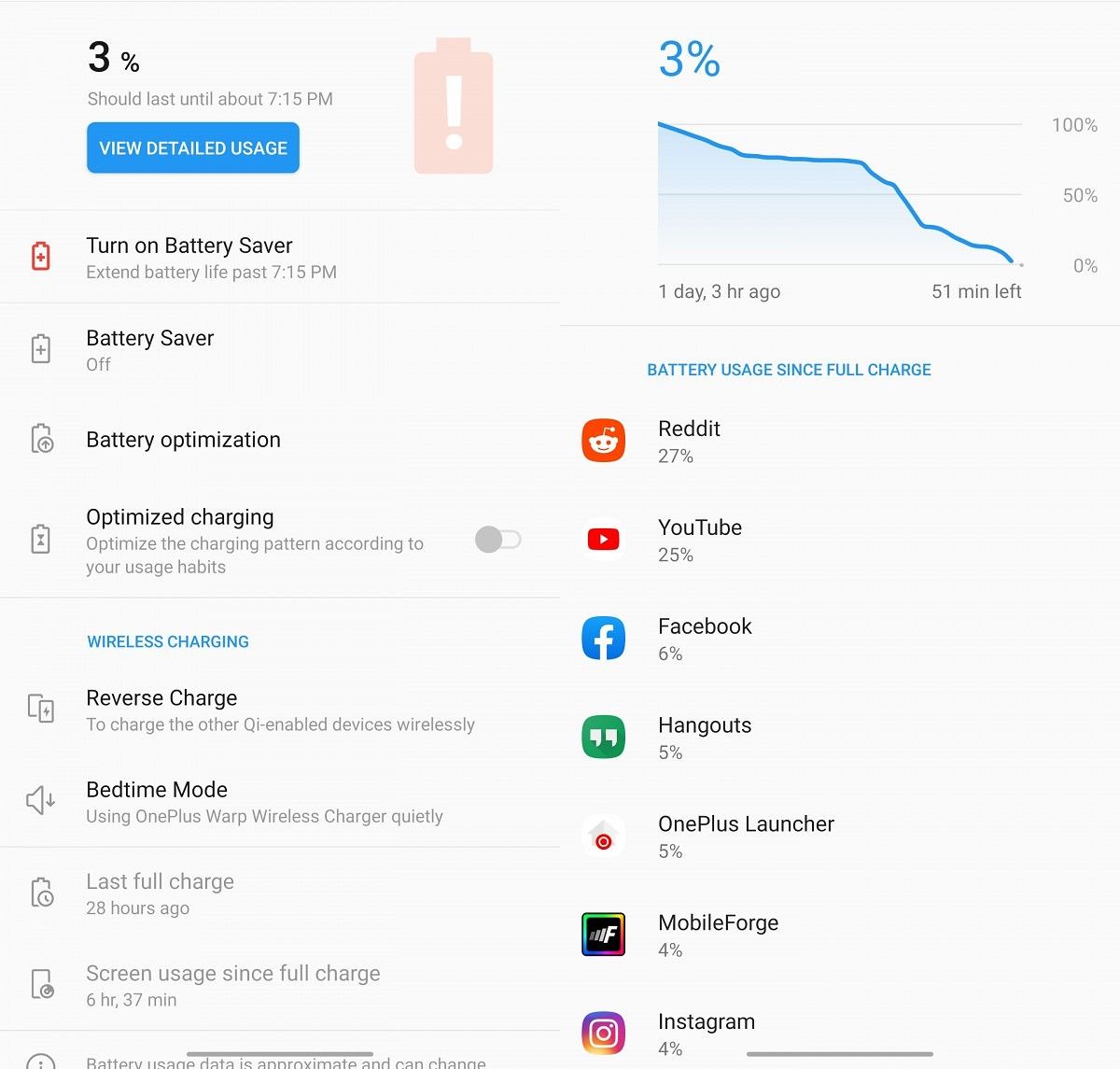Screenshot of a phone's battery settings screen displaying crucial information. At the top, the battery level is critically low at 3%, indicated by a battery icon and a note stating it should last until approximately 7:15 PM. A blue clickable box labeled "View Detailed Usage" is prominently featured.

Below this, options to extend battery life are presented. "Turn on Battery Saver" is suggested to prolong battery life beyond 7:15 PM, though the battery saver function is currently toggled off. The option for battery optimization, which aims to optimize the charging pattern based on usage habits, is also shown, and this feature is not activated.

A section with blue text titled "Wireless Charging" includes subcategories: 
- "Reverse Charge" which enables charging other QI-enabled devices wirelessly,
- "Bedtime Mode" for quiet charging using the OnePlus Warp Wireless Charger.
Additional information states the last full charge was 28 hours ago, with the screen active for 6 hours and 37 minutes since the last full charge.

A detailed battery usage chart is displayed on the right-hand side, indicating the current 3% battery level and illustrating the battery usage over the past day and three hours. The graph estimates 51 minutes of remaining battery life. 

Under "Battery Usage Since Full Charge," various apps and their battery consumption percentages are listed:
- Reddit: 27%
- YouTube: 25%
- Facebook: 6%
- Hangouts: 5%
- OnePlus Launcher: 5%
- Mobile Forge: 4%
- Instagram: 4% 

This detailed breakdown provides a comprehensive overview of the phone's battery usage and remaining lifespan.